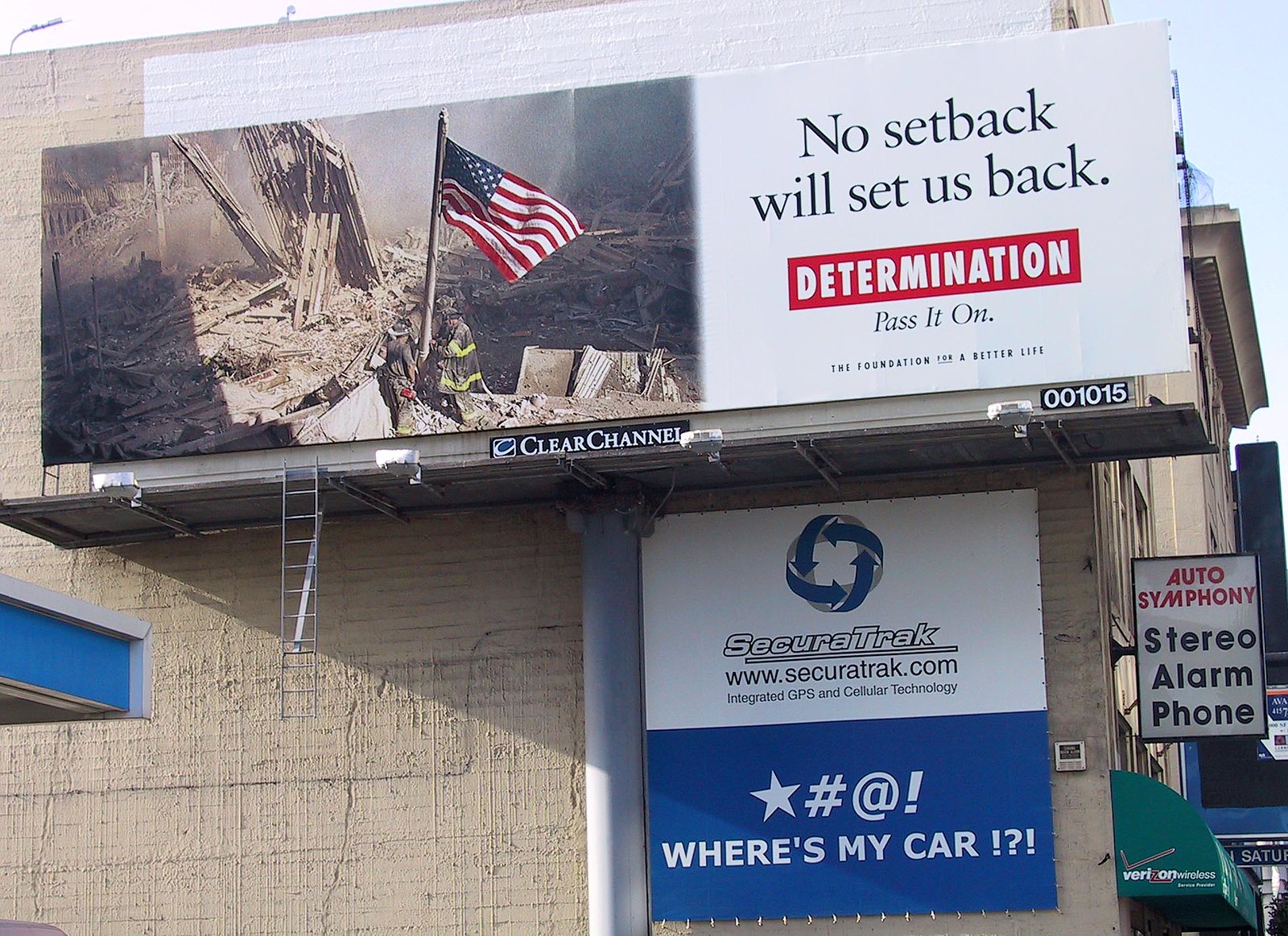This is an image of a corner building adorned with multiple signs and billboards. The most prominent feature is a large, horizontal billboard at the top, displaying a motivational message. The billboard depicts an American flag amidst rubble, reminiscent of post-9/11 scenes. The poignant message on the billboard reads, "No setback will set us back," with the word "Determination" highlighted in red. Below this, it says, "Pass it on - The Foundation for a Better Life." The billboard, identified as Clear Channel 001015, emphasizes resilience and determination.

Directly beneath this motivational billboard is a smaller sign advertising Secure Track, complete with a web address, www.securetrack.com, and the tagline "Where's my car," hinting at a GPS and cellular tracking service.

Adjacent to these, on the front side of the building, there is a vertical sign for "Auto Symphony," advertising services related to stereos, alarms, and phones. Additionally, one of the building's awnings prominently displays the logo of Verizon Wireless, indicating the presence of a phone store.